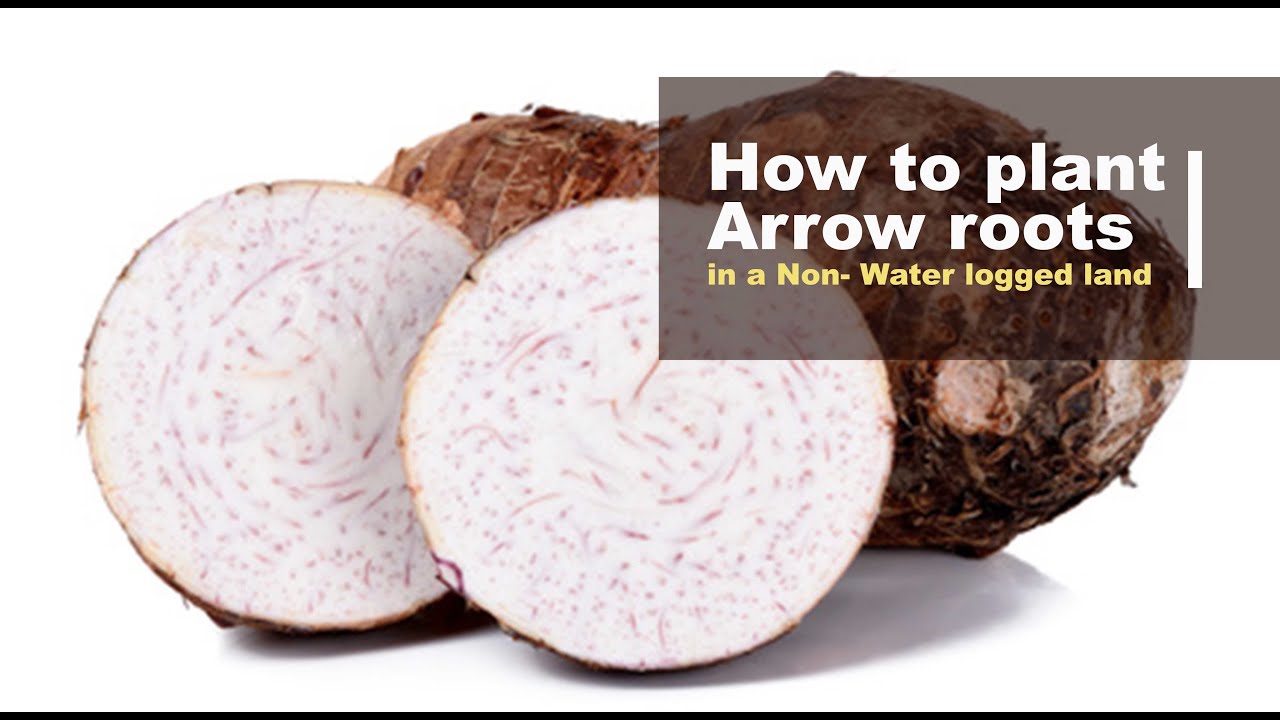The image depicts a close-up view of arrow roots, prominently featuring a root that is split open to display its intricate interior. The cross-section reveals detailed differentiation between the inner and outer parts: inside, there are swirling brown lines amidst a primarily white core, while the exterior skin is a dark brown. Additional whole and cut segments of the root are visible, giving a comprehensive view of the plant. The setup is centered against a stark white background, possibly taken in a light box, with clear visual emphasis on the root's details.

Framing the illustration are two horizontal black lines at the top and bottom of the image. In the top right corner, a gray, translucent text box overlays part of the root, containing white and yellow text that reads, "How to Plant Arrow Roots in a Non-Waterlogged Land." This aesthetically arranged composition suggests that the image is designed for an educational context, such as a website or a how-to guide, offering viewers detailed visual and textual information on arrow roots.